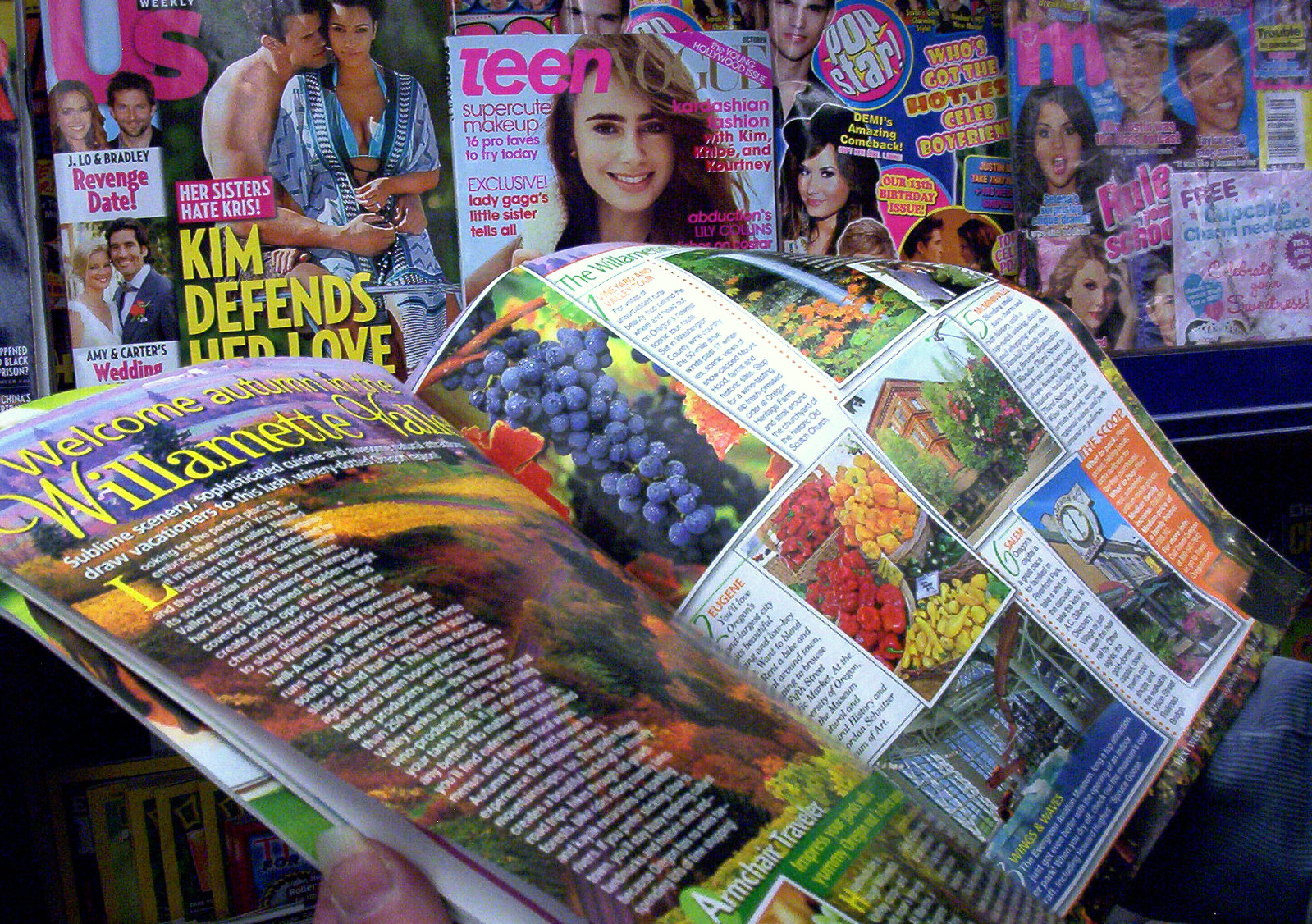In this image, a person is holding an open magazine, showcasing vibrant, multicolored pages filled with detailed photographs and text. The focal page features "Willamette" prominently, with rich images of grapes, baskets of fruit, and assorted vegetables including red peppers, suggesting a theme related to wine country or autumn harvest. In the backdrop, various popular magazines such as Teen Vogue, Popstar, and Us Magazine with headlines like "Kim Defends Her Love" featuring Kim Kardashian can be seen neatly arranged on a magazine stand. The setting appears well-lit, possibly indicating an indoor environment, such as a bookstore or a newsstand, with a blue frame giving structure to the stand full of periodicals.